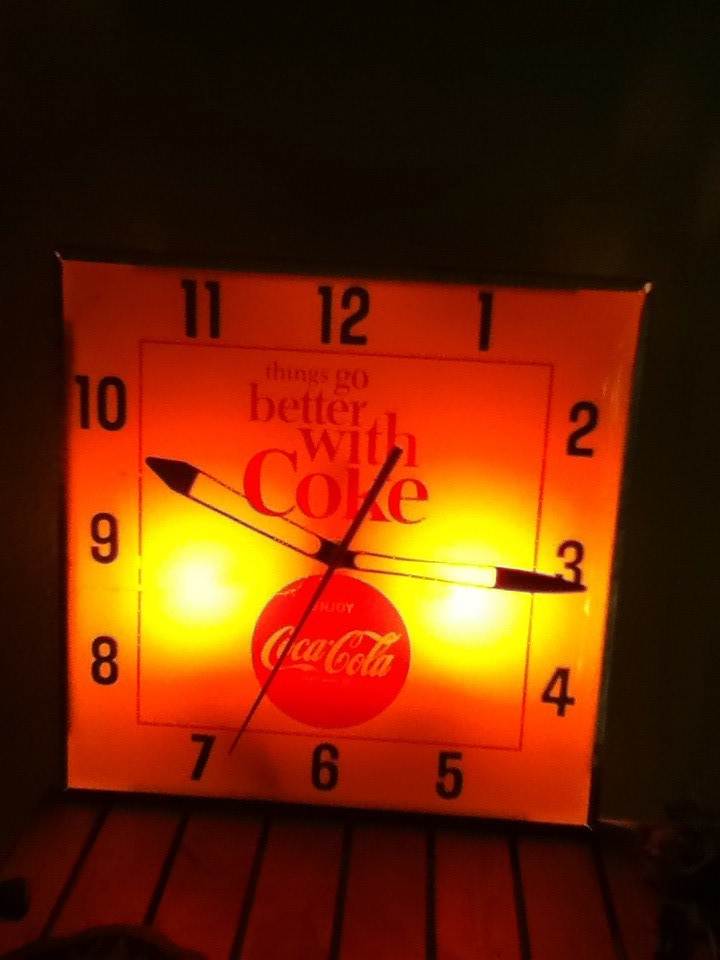The image depicts a close-up of a square Coca-Cola branded clock positioned on wooden floor planks in a dimly lit room. The clock face is illuminated from behind by warm white lights on either side, casting a soft glow. The clock's white face contrasts with its black hands and numbers, and prominently features the iconic Coca-Cola logo at the bottom. Above the logo, the slogan "Things Go Better With Coke" is clearly visible. The clock currently displays a time, which varied in the descriptions, but notably mentions points around 9:16, 10:15, and 3:50. The overall color tone of the illuminated clock face is a mix of warm and red hues, adding a nostalgic ambiance to the scene.